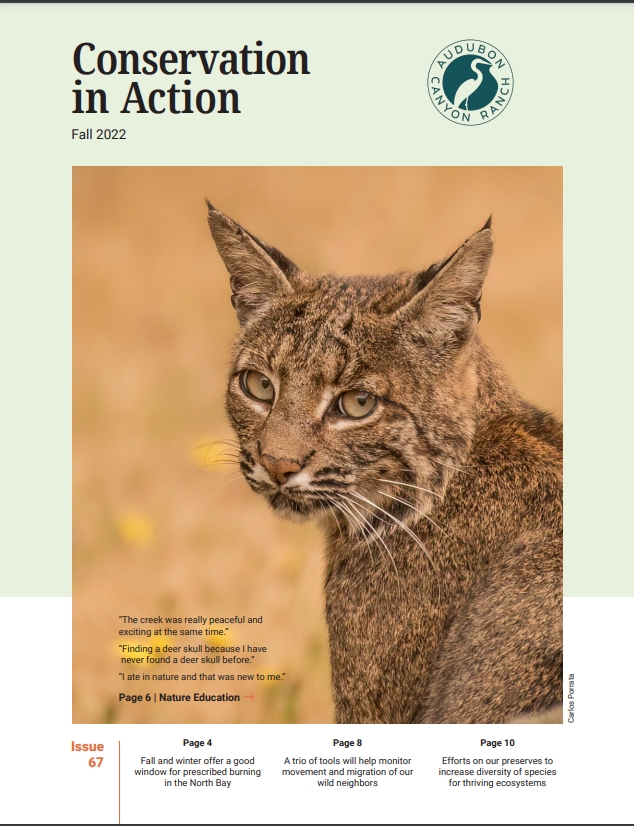The cover of the Fall 2022 edition of "Conservation in Action," published by Audubon Canyon Ranch, features a striking photograph of a wild bobcat. The bobcat, with its intricate patterns and multi-colored markings, stands against a blurred pinkish-beige background, turning its head to look directly at the viewer. Every detail is captured in high focus, showcasing its whiskers, golden brown eyes, and alert ears. The Audubon Canyon Ranch logo, depicting an egret within a green circle, sits in the upper corner alongside the title. The issue, labeled as Issue 67, includes various educational insights, with teasers for articles such as prescribed burning in the North Bay on page 4, tools for monitoring wildlife migration on page 8, and efforts to increase species diversity on page 10. Additionally, quotes about engaging with nature, from peaceful creek experiences to finding a deer skull, highlight the publication's theme of immersive nature education, referenced on page 6.